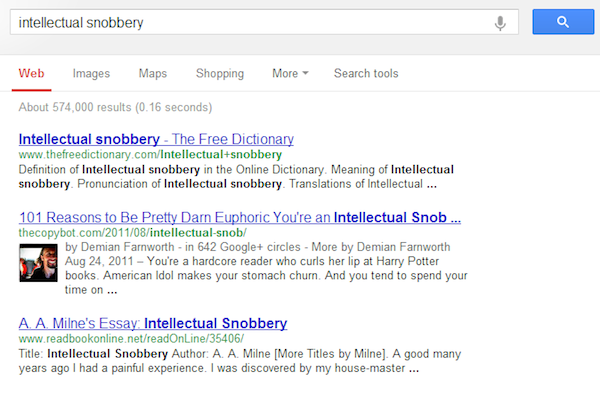Here is a detailed, cleaned-up caption based on the provided description:

---

The image features a Google search results page with "intellectual snobbery" entered into the search bar, which is displayed as a gray bar. To the left of the search bar, there's a microphone icon, and adjacent to it is a search button. Below the search bar, six tabs are visible: Web, Images, Maps, Shopping, More, and Search Tools.

On the left side, there's an icon resembling a web with a red LED indicator. The search results are displayed below this, showing three different posts. 

1. The first result is titled "Intellectual Snobbery" from The Free Dictionary, with the corresponding web address listed below it, followed by a brief description of the content.
2. The second result is an article titled "101 Reasons to Be Pretty Damn Euphoric: You're an Intellectual Snob" with its website, followed by a short summary underneath.
3. The third result is an "AA Mind Essay" on Intellectual Snobbery, also featuring its web address and a brief description below.

This detailed view provides a clear snapshot of the top results for the query "intellectual snobbery," showcasing the variety of interpretations and discussions available online.